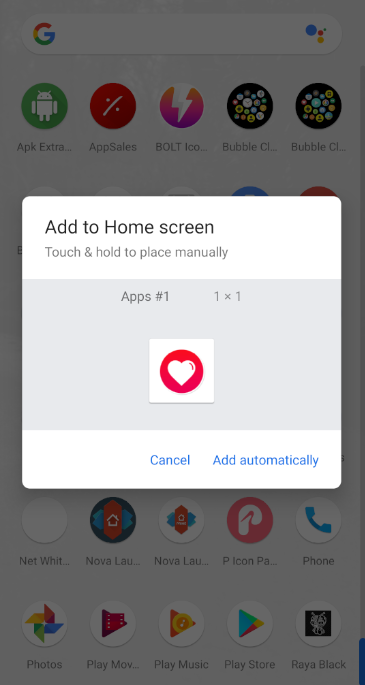A colorful and vibrant splash screen displaying various app icons and descriptors. Prominently featured are:
1. The APK extra icon: a green circle with a white robot.
2. The App Sales icon: a red circle with a tilted division symbol.
3. The BOLT icon: capitalized letters "B-O-L-T" over a rainbow background blending purple, pink, and orange, with a white thunder symbol.
4. An icon with clouds labeled "C-L", accompanied by two similar icons with colorful bubbles.

The screen has a white square overlay containing:
1. "Add to Home Screen" instructions.
2. "Touch and hold to place manually" directive.
3. An apps panel showing “pounce” icon sized at 1x1.
4. An option panel with "Cancel" and "Add Automatically" buttons in blue, housing a white square with a red heart.

In the background, beside the overlay:
1. Several app icons including one with "W-H-I-T."
2. The Nova Launcher logo, partly obscured.
3. A blue circle with an orange stripe, topped by a white hat.